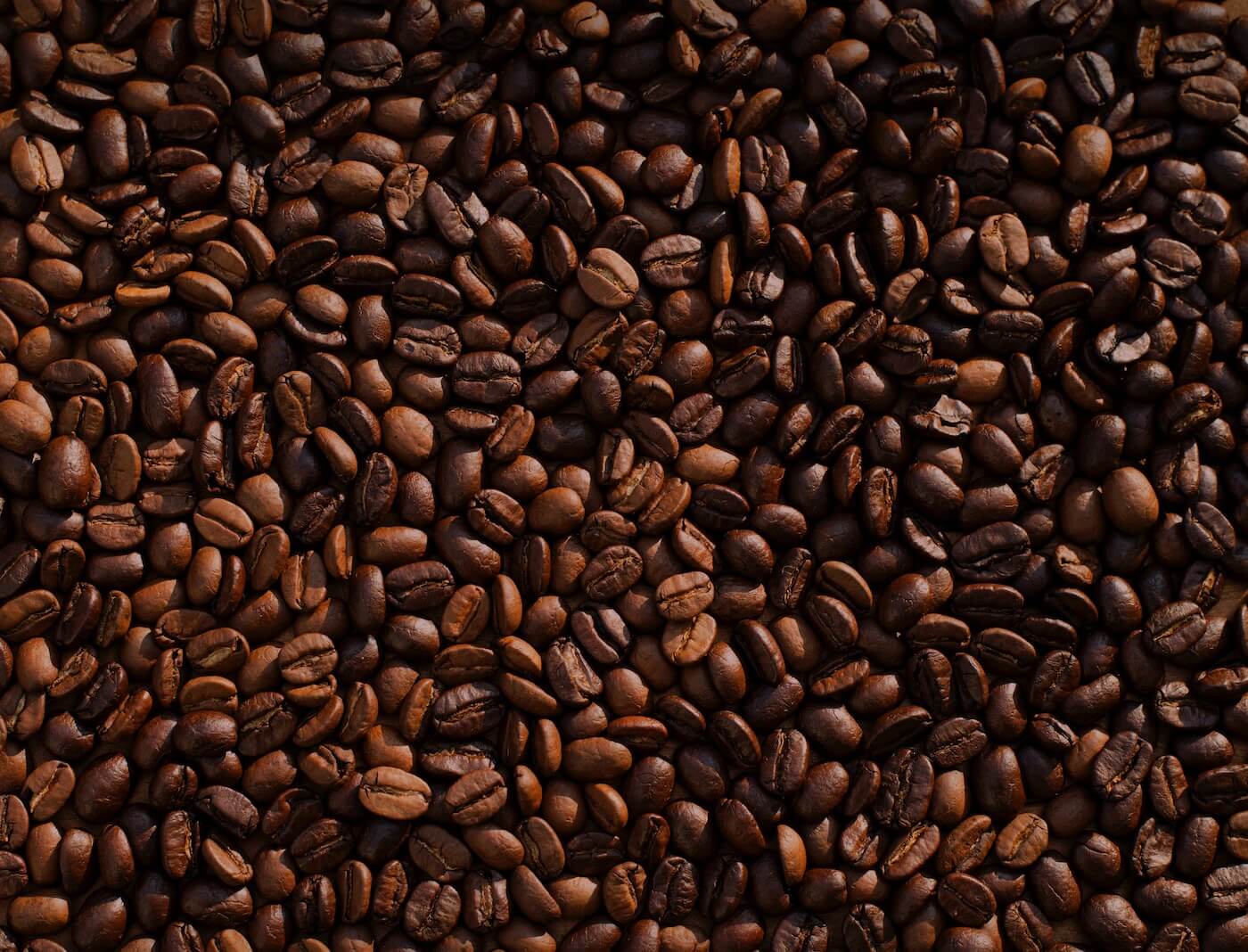This top-down photograph captures hundreds, if not thousands, of roasted coffee beans filling the entire frame. The beans vary widely in texture and shading, showcasing a spectrum of browns from pale to very dark. Some beans prominently display their characteristic central crease, while others show their smooth, rounded backs. The lighting, which appears to come from different sources, creates intricate highlights and shadows across the image. This interplay of light causes some areas, particularly the top and the right sides, to feature darker beans, while the bottom and the left sides reveal lighter shades. The beans are not arranged in any particular pattern, simply scattered naturally, enhancing the sense of randomness and realism in the composition.